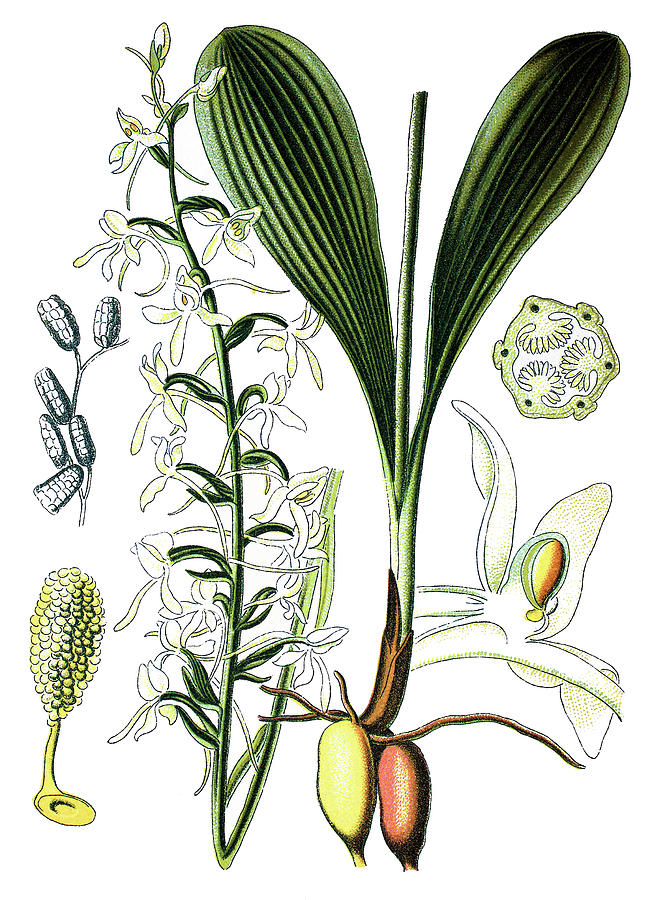This illustrated image features various detailed parts of different plants displayed on a plain white background. Central to the image is a green plant with very long leaves and a plain stem, deeply rooted with nodules near the roots. Beneath these roots are yellow and orange oval objects, outlined in brown. To the left of the main plant is a long-stemmed plant adorned with small, white flowers spaced approximately half an inch apart along its stem. Further on the left, a yellow corn-like flower is depicted, as well as a purple-toned plant. In the bottom left corner, a segment presents a honeycomb dripping honey into a puddle. Adjacent images showcase various plant parts, including a detailed yellow flower center with small yellow balls and another black and white depiction showing buds, and textured circular images. On the right side of the illustration, a seed-like flower and a large white standalone flower are shown, contributing to the diverse representation of plant anatomy in this comprehensive illustration.